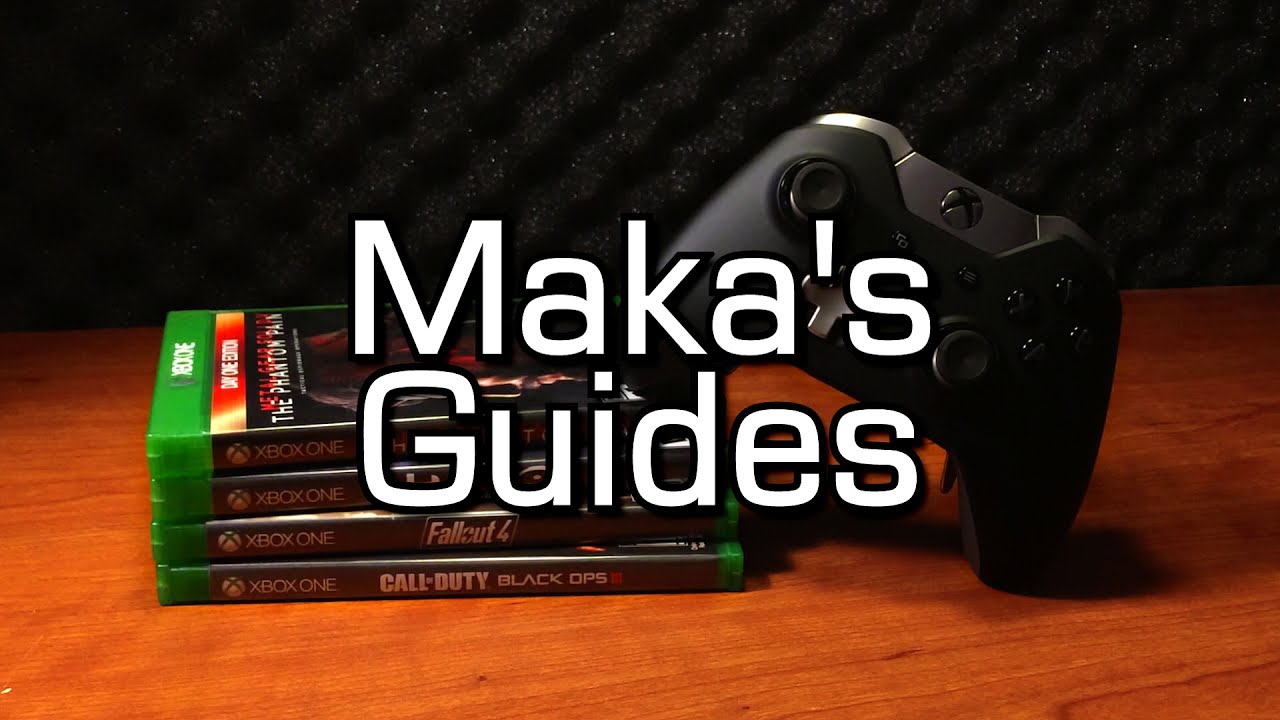The image is a professionally shot, digitally enhanced horizontal banner or YouTube thumbnail depicting a neatly arranged scene. It features a medium brown wooden desk set against a black background, which appears to have a cushiony, sound-dampening material, ideal for acoustics. On the desk sits a stack of four Xbox One video game cases. The clearly visible titles are Call of Duty Black Ops at the bottom and Fallout 4 above it, while the titles of the top two games, including a partially discernible Metal Gear Solid: The Phantom Pain, are obscured. Resting diagonally on top of the game cases is a black Xbox One controller, propped to face the viewer. In the foreground, large white text overlay reads "MACA'S GUIDES," contributing to the impression that this image is intended for a blog or video content, possibly tutorial or review-based. The setup benefits from precise, professional lighting, casting appealing shadows that give the scene depth and clarity.